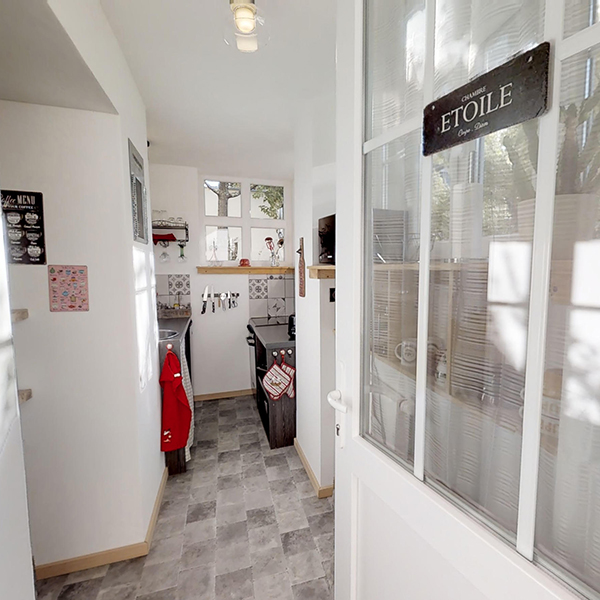This image captures the view through a white glass-paneled door, adorned with a black sign reading "Etoile," into a meticulously organized kitchen area. The doorway, open on the right, frames a clean and inviting culinary space. The kitchen floor is tiled, and the color scheme spans white, yellow, pink, black, gray, and red, lending a vibrant yet cohesive atmosphere. On the left, a silver countertop with a sink is visible, whereas on the right, another silver countertop with a black oven beneath has oven mitts hanging nearby. The back wall, mostly white, features a window with a tan wooden shelf below it. Above the countertop is a magnetic knife strip. The walls showcase various hanging items and art, adding to the kitchen's charm and neat organization.